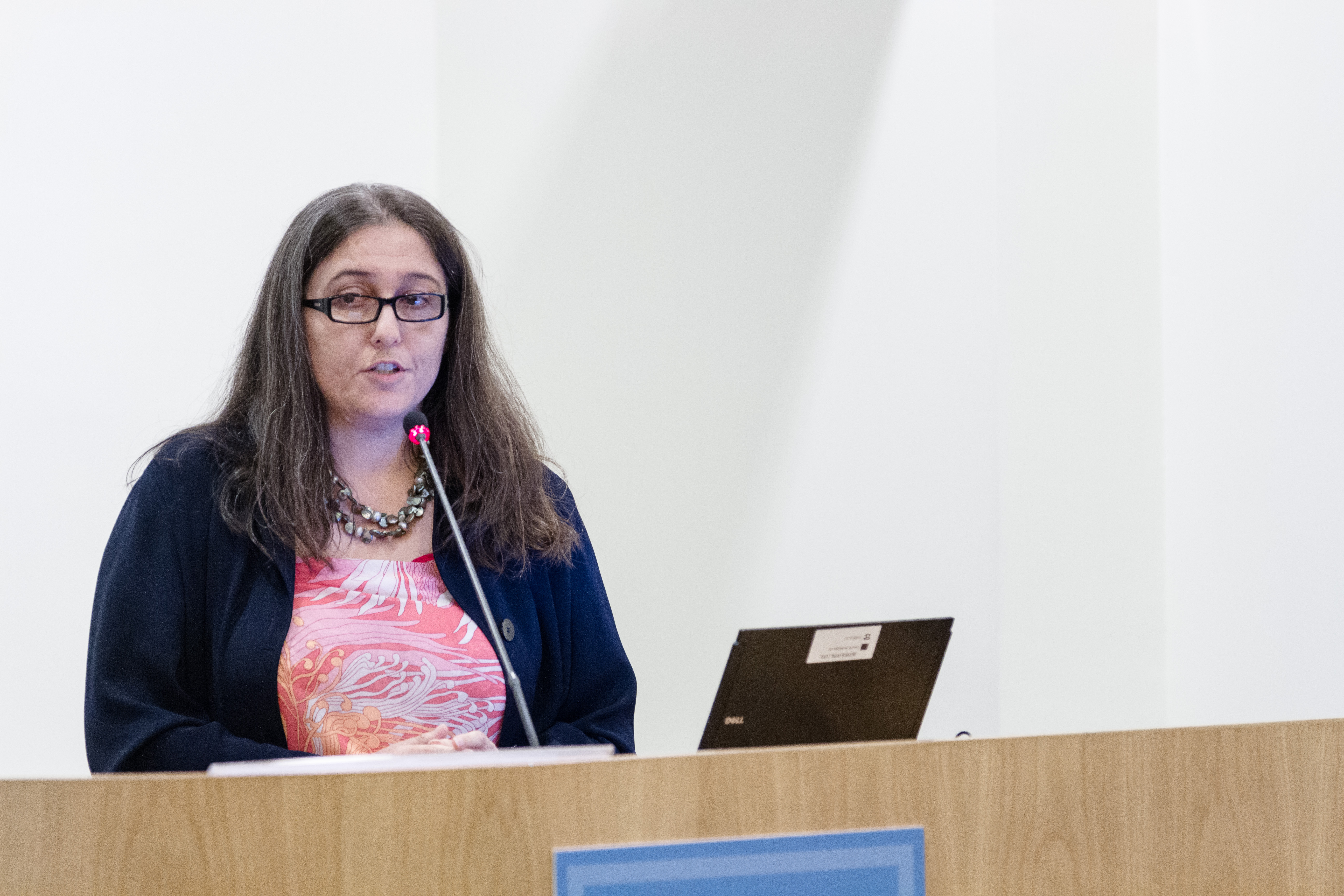A woman is giving a speech or lecture behind a large, light tan wooden podium in a modern, mostly white auditorium. She appears to be a college professor or speaker, talking into a long silver microphone. She has shoulder-length, slightly wavy, and somewhat messy brown hair, wearing black rectangular glasses. She is dressed in a blue cardigan over a red dress and accessorized with two bead necklaces. Her fair-skinned, round face shows her in mid-speech, looking slightly to her right. The podium also holds an open laptop. The background is stark white, emphasizing the modernist and possibly an academic setting, though no audience is visible in the photograph.